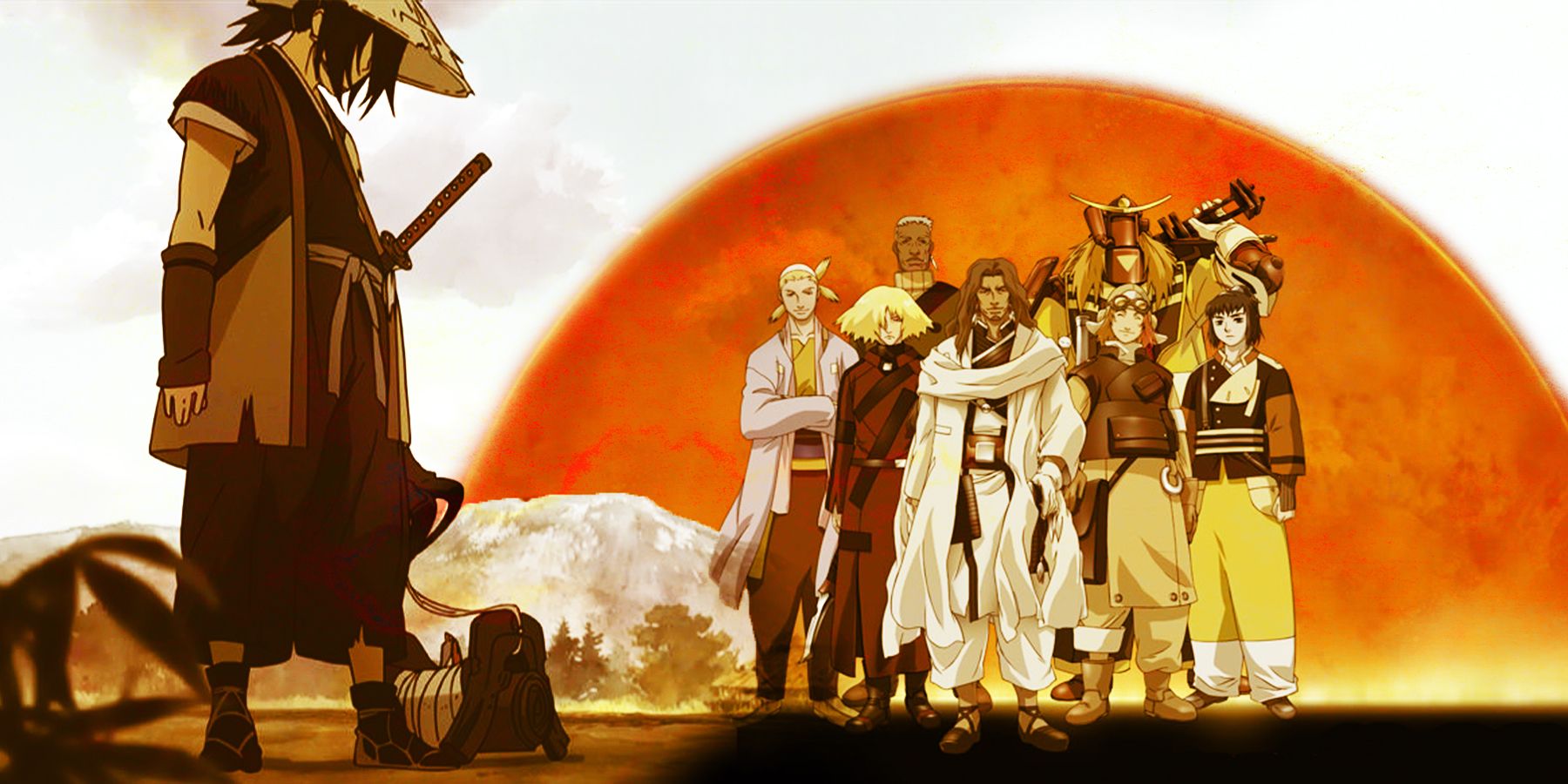The anime-style image depicts a dynamic scene just right of center, showing a diverse crowd of seven people standing and facing forward. Among them, a colossal metal figure with a sword strapped to his back stands prominently. The group features individuals adorned in varied attire: a man donning white, flowing robes; another in red and black robes; and a person with goggles perched on their forehead, suggesting a mix of different backgrounds, skin colors, and genders.

Behind the group, a striking orange sun looms on the horizon, casting an evocative light across the scene. To the left, distant mountains create a serene backdrop. Closer to the foreground on the left, a solitary character, perhaps a ninja or warrior, stands wearing a traditional conical Asian rice hat made of grass. This figure, cloaked in a brown robe, has long black hair that partially obscures his face and a sheathed sword at his side, his gaze directed downward towards the ground.

Overall, the scene combines varied elements from Japanese culture, including references to samurai and ninjas, to create a rich and evocative tableau of characters set against a dramatic, sunlit landscape.